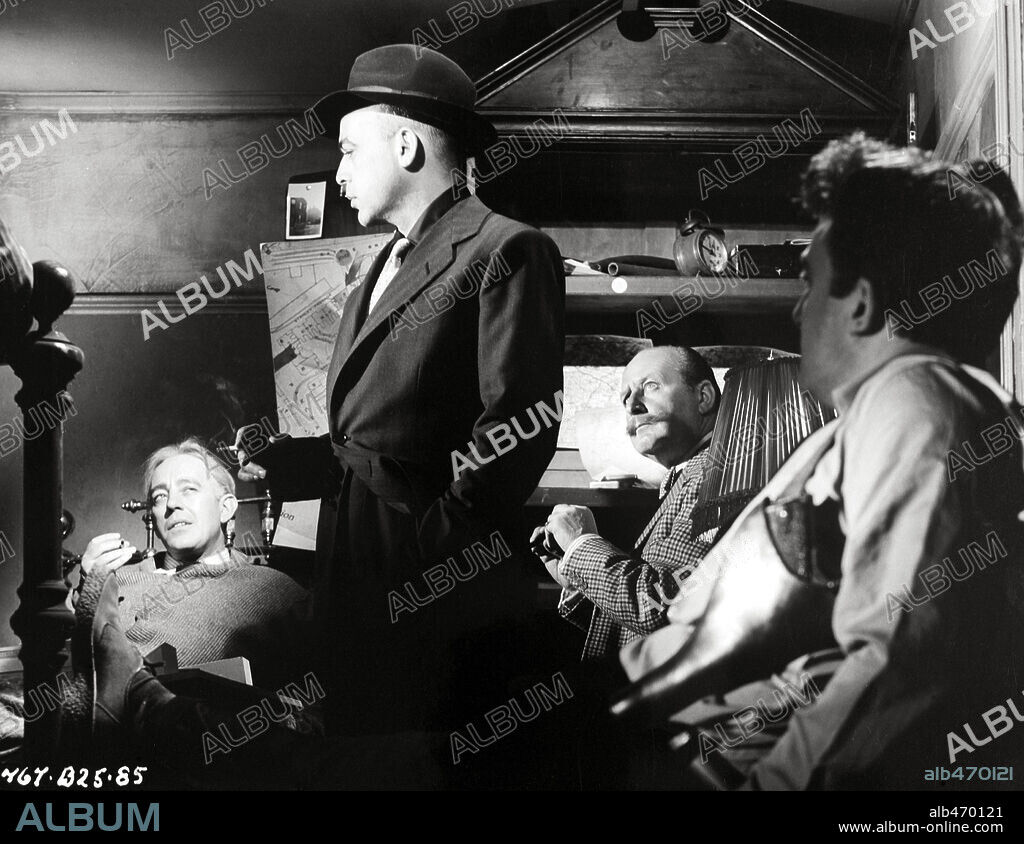This black and white photograph, possibly from the 1930s or 1940s, features an indoor scene with significant vintage elements such as wooden paneling and ornate furniture. The setting appears to be an office or perhaps a set for a movie or play. There are four men in the picture: one man in his 50s, wearing a sweater, is sitting on the left and looking up at another standing gentleman. This standing man, dressed in a black suit and hat, possibly a bowler, is smoking a cigarette and looking off to the side. Another man, also in his mid to late 50s with a large mustache and balding, is seated behind the standing man and also looking up at him. In the foreground, to the far right, a fourth man is partially visible, with only a third of his face shown as he is turned away, directing his attention towards the man with the hat. The background features a wind-up alarm clock on a shelf alongside some records or knickknacks pinned to the wall, and possibly a map or photographs. The image has a watermark saying "Album" across it and a URL www.album-online.com in the lower right corner, indicating it is a stock photo from a company named Album.